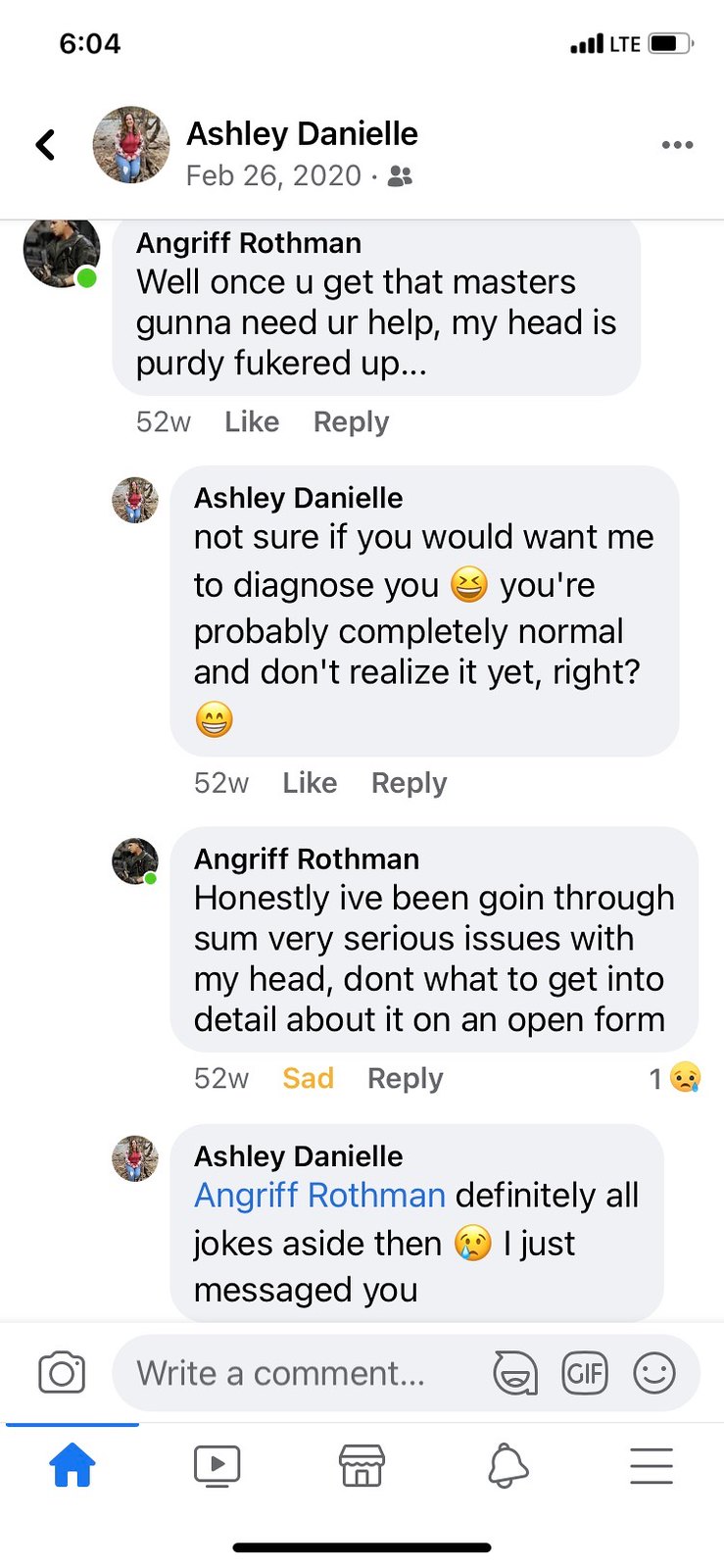The image is a detailed screenshot of a text conversation between two individuals on a social media platform, likely resembling Facebook Messenger. At the top left corner, the time reads 6:04, while the right corner displays phone information, including an LTE signal and a battery indicator showing approximately 70% charge. The main header features "Ashley Danielle" with her profile picture and the date, February 26, 2020, right below her name.

Ashley Danielle initiates the conversation, and the text bubbles are color-coded in gray. She is pictured in a profile image wearing a red shirt and blue jeans, sitting in front of a tree with dirt around, hinting at an outdoor setting. The conversation unfolds as follows:

1. Angriff Rothman writes, "Well, once you get that master's, gonna need your help. My head is pretty fuckered up."
2. Ashley Danielle responds with, "Not sure if you would want me to diagnose you. You're probably completely normal and don't realize it yet, right? :)"
3. Angriff Rothman replies, "Honestly, I've been going through some very serious issues with my head. Don't want to get into detail about it on an open forum."
4. Ashley Danielle then sends a sad face emoji and follows up with, "Angriff Rothman, definitely all jokes aside then, I just messaged you."

At the bottom of the image, there are input fields and icons for adding comments, alongside symbols for a home button, video, and notifications, further suggesting it is a mobile interface capturing real-time text interactions.